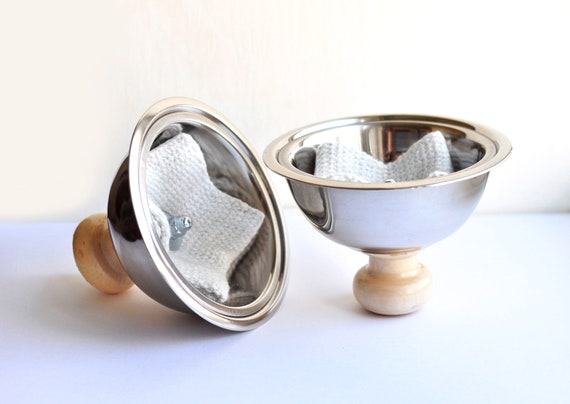This color photograph features two metallic, bell-shaped objects placed on a bluish-colored tabletop with a white wall behind them. Both objects have a light-colored wooden handle, screwed into the apex of a silver metal bowl. The handles are knob-shaped and taper towards the base. The left object is oriented upright, revealing the inside of the bowl which contains a piece of white fabric. The right object is upside down, with the handle positioned at the bottom, also showing the fabric within the bowl. The overall appearance suggests these could be covers or lids, such as for a sugar container or salt and pepper shakers.